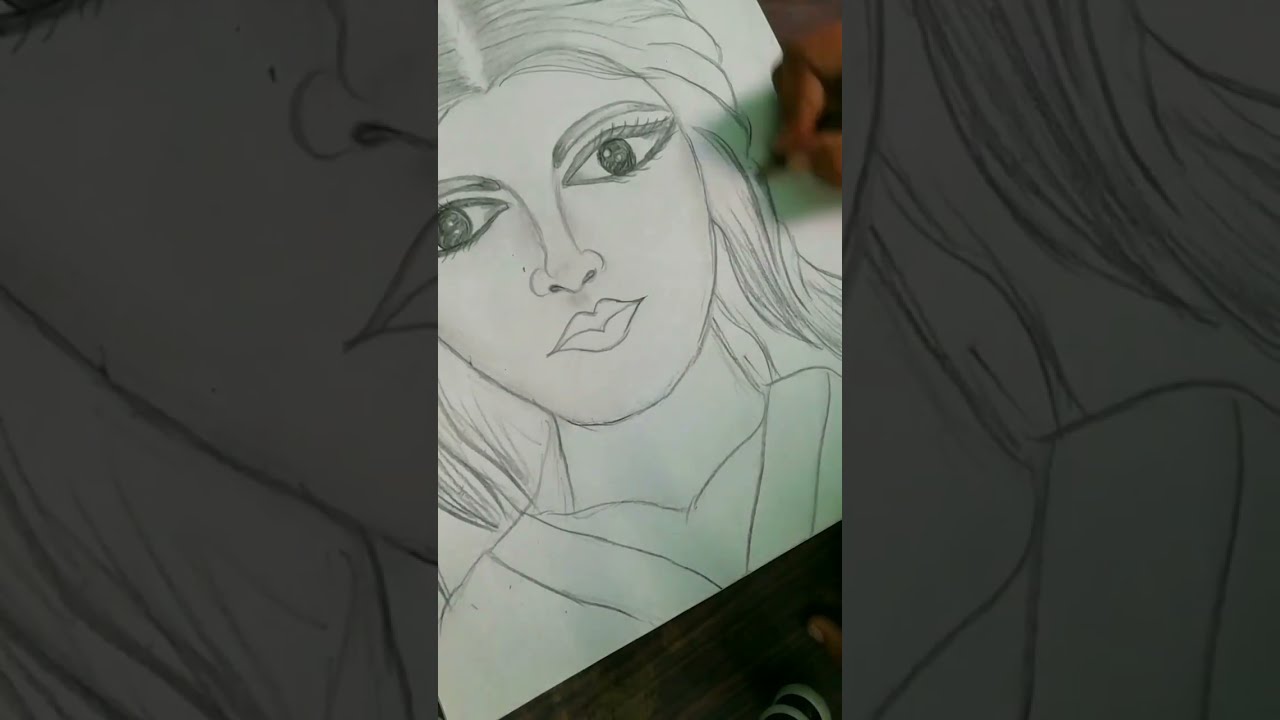This image is a wide rectangular composition featuring three sections. The central section showcases a pencil drawing on white paper, turned slightly diagonal to the left. The drawing depicts a woman with large, expressive eyes and long, thick, straight hair parted in the middle. She has a small, pointy nose, lips shaped like a heart, and very long, thick eyelashes. She is wearing a V-neck top, possibly layered or with intricate detailing. The woman's shoulders are visible, highlighting her upper body, and a blurry hand is noticeable in the top right corner, suggesting the act of drawing. Flanking the central drawing, the left and right sections display slightly shaded, blown-up close-ups of parts of the drawing, emphasizing the hair and facial features on the left and more hair along with the shoulder on the right. The overall composition gives a detailed, magnified view of the pencil drawing while maintaining focus on the central image of the woman.